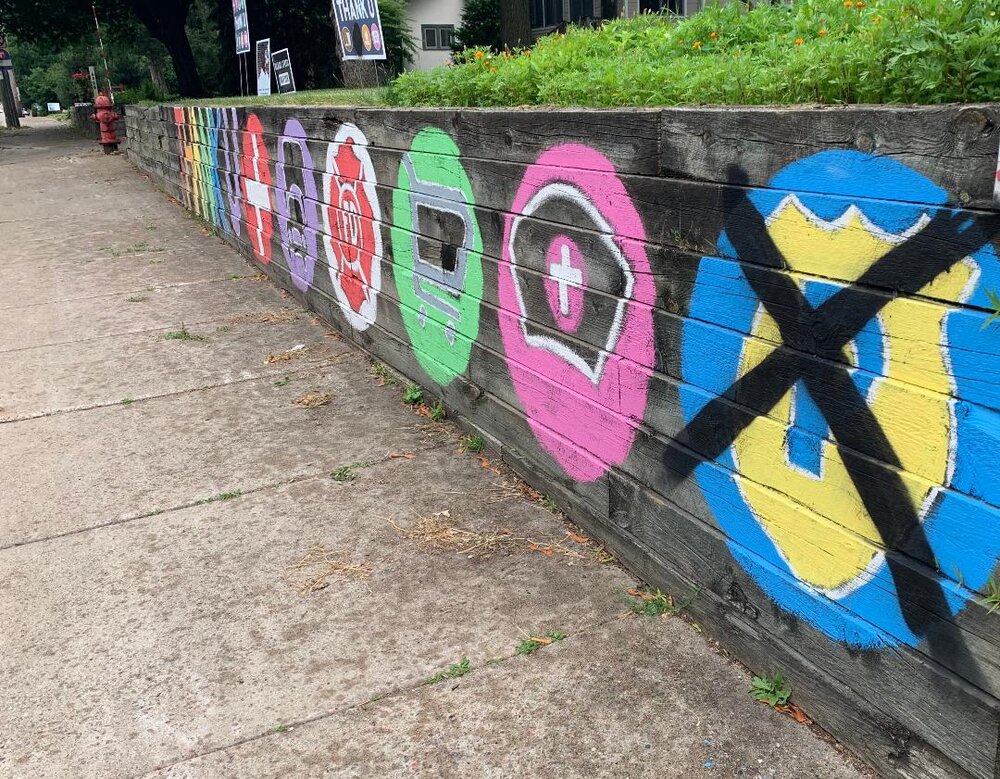This photorealistic outdoor image captures a wooden retaining wall adorned with a series of colorful, circular paintings viewed from a sidewalk. The wall, extending alongside a yard with some grass or weeds and sprouting orange flowers from its top, displays various vibrant circles each containing distinct illustrations. In the first blue circle closest to the foreground, there is a yellow police badge with a blue 'P' in its center, crossed out by a black 'X'. Following this are multiple other circles: a violet one with a black shield outlined in white, containing a smaller violet circle and a white cross in its center; a green circle featuring a grey shopping cart; a white circle with an unreadable red design; and an additional violet circle with an indistinct black image. Other circles along the wall involve multiple colors including violet, blue, green, yellow, and pink, with some letters that are not readable due to the viewing angle. Toward the far end of the wall stands a red fire hydrant, and behind the wall, there are trees and signs posted in the neighboring yard.